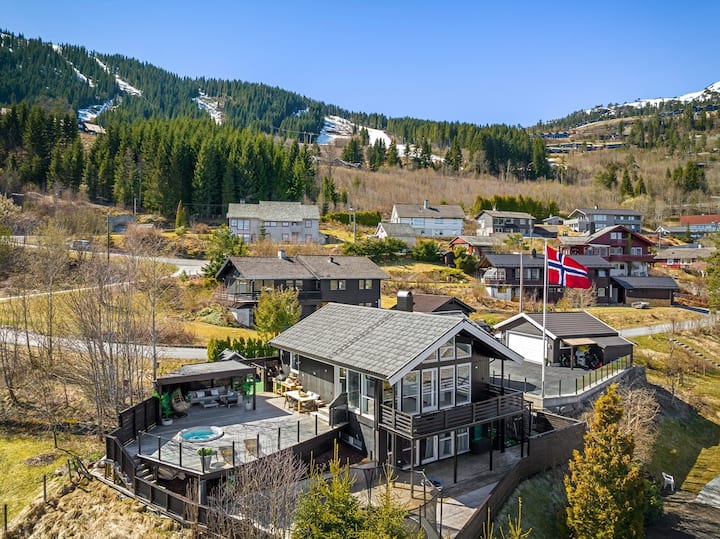This vibrant color photograph captures a picturesque neighborhood nestled on a large hillside, with a striking backdrop of towering snow-capped mountains and an expansive blue sky. The focal point is a distinctive two-story black house with extensive white-framed windows adorning the entire front facade. This house features a spacious balcony porch and a sizable deck on the side, which includes a covered area with a swing, an egg chair, and various plants. An inset hot tub enhances the deck's appeal, while stairs lead down from it. The property is enclosed by a black privacy fence and displays a flagpole flying a Norway flag. Adjacent to the house is a matching garage.

Beyond this prominent house, a mix of brown, tan, and white houses is scattered up the hillside, connected by asphalt roads. A driveway and secondary patio are also visible from the primary house. The scene is rich with lush greenery and an abundance of conifer trees. Paths weave through the landscape, adding to the serene and verdant atmosphere. This idyllic hillside community appears meticulously maintained, with neatly kept grass and a multitude of trees enhancing its rural charm.